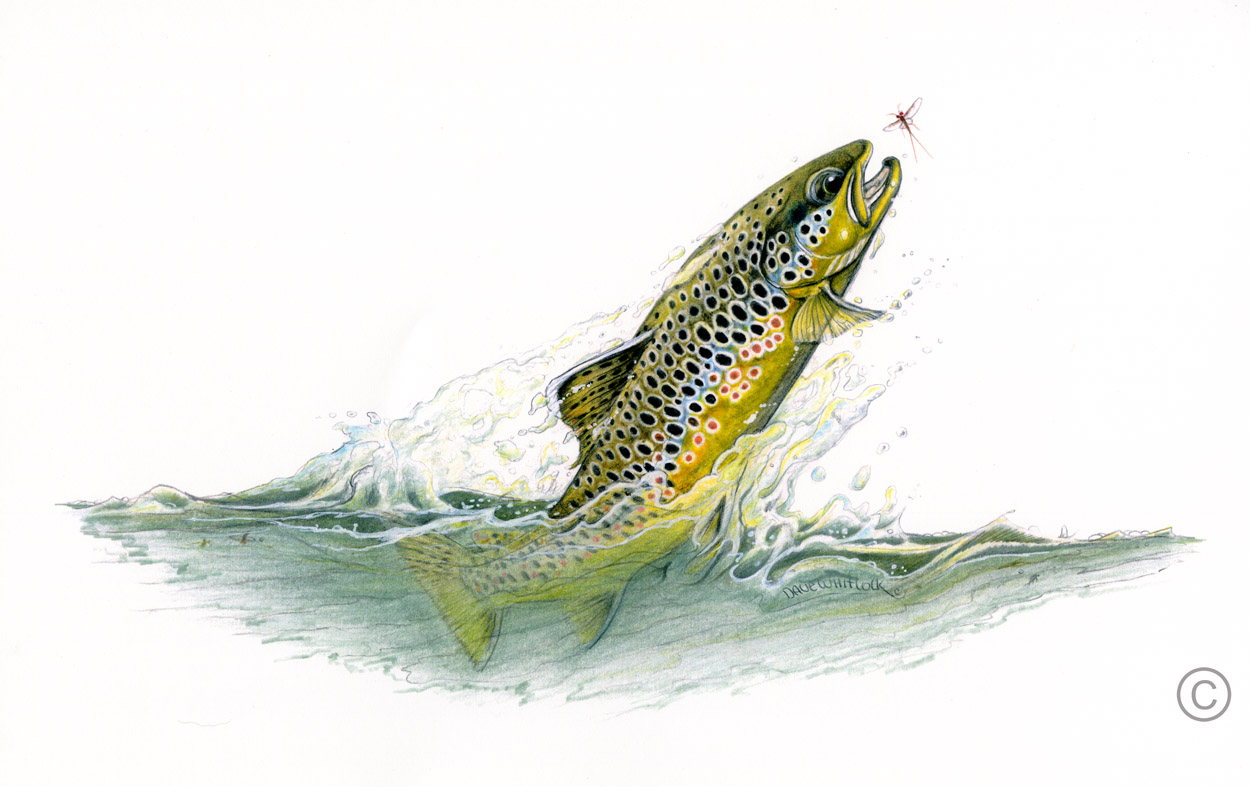This detailed painting, created by Dave Whitlock, captures a vivid scene of a fish leaping out of greenish water to catch a dragonfly. The fish's body is mostly above the surface, with its vibrant yellow color adorned by black and red spots. Its head and upper body exhibit shades of dark to light green, marked by black dots outlined in white. The fish’s eye is detailed with a black circle and a white dot in the center. Below the water, the artist’s signature is visible. The water, depicted in various shades of green and blue, has subtle waves forming an arch shape as it splashes around the fish. The dragonfly, poised above, features a long purple and blue body, red eyes, two black wings, and a forked tail with two legs extending backward. The painting's background is white, framed in a horizontal rectangular shape with a copyright symbol at the bottom right corner.